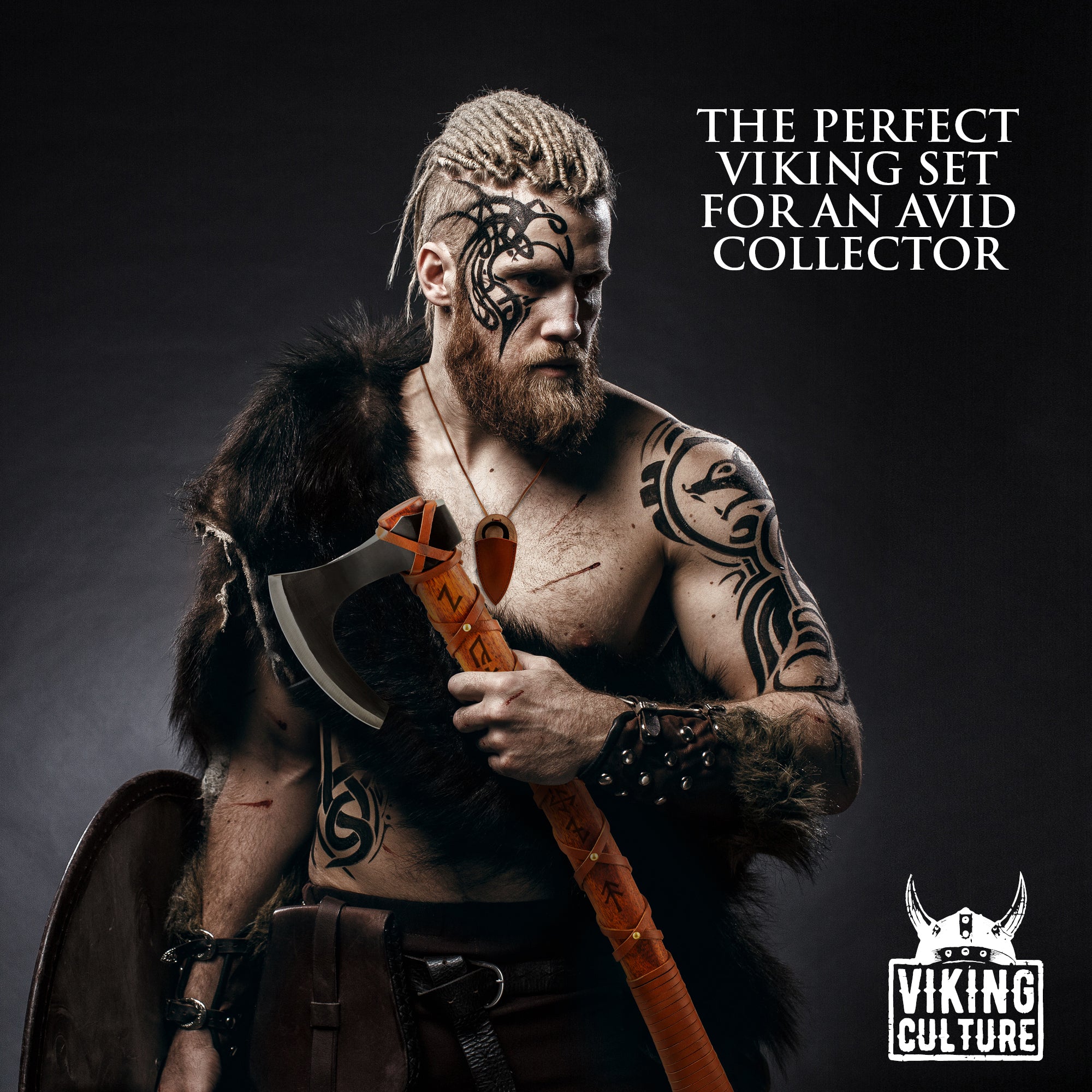This advertisement features a striking image of a man posed against a solid black background with slight light illumination from the bottom left. Central to the frame is a white man with blonde dreadlocks, half of his head shaved, and a full beard. His face and arms are adorned with sharpie-drawn tribal tattoos, including a squirrel-like design on his forehead and cheek, and what seems to be a dragon tattoo on his left arm.

Dressed in authentic-looking Viking attire, he sports a fur panel on his left shoulder and a brown leather skirt fastened by a black belt, which also holds a brown pouch. In his left hand, he grips an intricately wrapped leather axe with symbols etched onto it; the axe itself has a reddish-brown handle and a black blade with a silver streak. His right arm, which boasts additional tattoos, is equipped with a metal shield strapped to a panel guard that covers his wrist and forearm. 

The text "The Perfect Viking Set for an Avid Collector" is prominently displayed in white in the top right corner. At the bottom right, encased in a white-outlined box featuring a Viking helmet with horns, is the phrase "Viking Culture," adding an authentic touch to the advertisement.